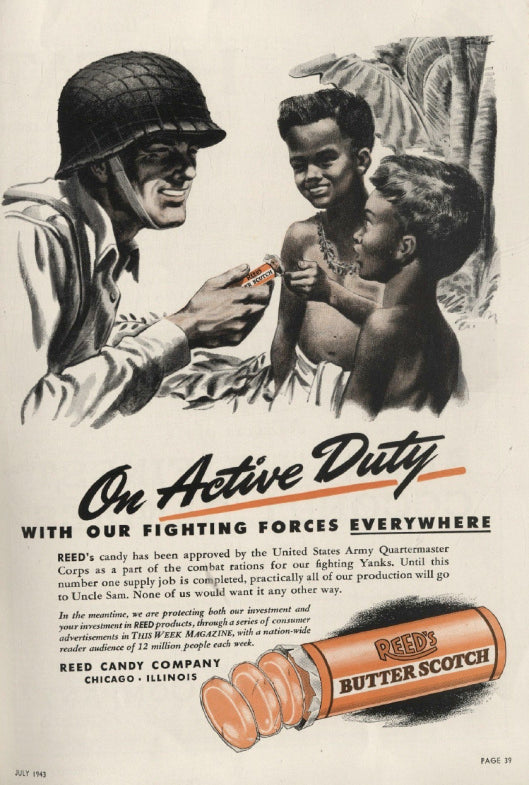This vintage advertisement for Reed's Butterscotch depicts a G.I. soldier in an old-style army helmet, smiling and extending a pack of the candy to two dark-skinned boys. The scene hints at a tropical setting, indicated by palm trees in the background, possibly evoking the atmosphere of the Vietnam War era. The boys, one wearing a toga-like garment and the other bare-chested, appear on an island, further emphasizing the exotic locale. The advertisement, laid out like a magazine page, features the bold headline "On active duty with our fighting forces everywhere." A textual section below elaborates that Reed's Butterscotch has been approved by the United States Army Quartermaster Corps as part of combat rations, reinforcing the idea that the candy plays a supporting role in the soldiers' daily lives. The message concludes with a patriotic note about the priority being given to Uncle Sam's needs.